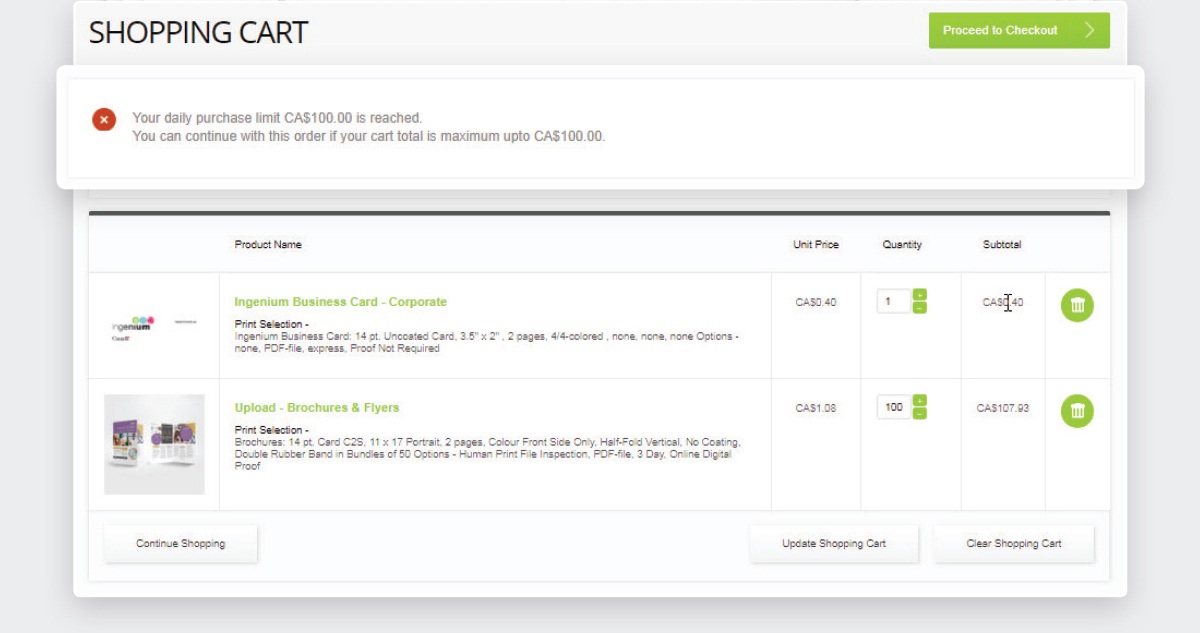A minimalistic online shopping cart interface displays two items related to business office supplies. The first item is an "Ingenium Business Card-Corporate" in a quantity of one. The second item is "Upload Dash Brochures and Flyers" with the quantity set to one hundred. All prices appear to be in Canadian dollars. An error message at the top indicates that the total order exceeds the daily purchase limit of one hundred Canadian dollars, suggesting the shopper needs to reduce the quantity of the brochures and flyers to proceed with the order.